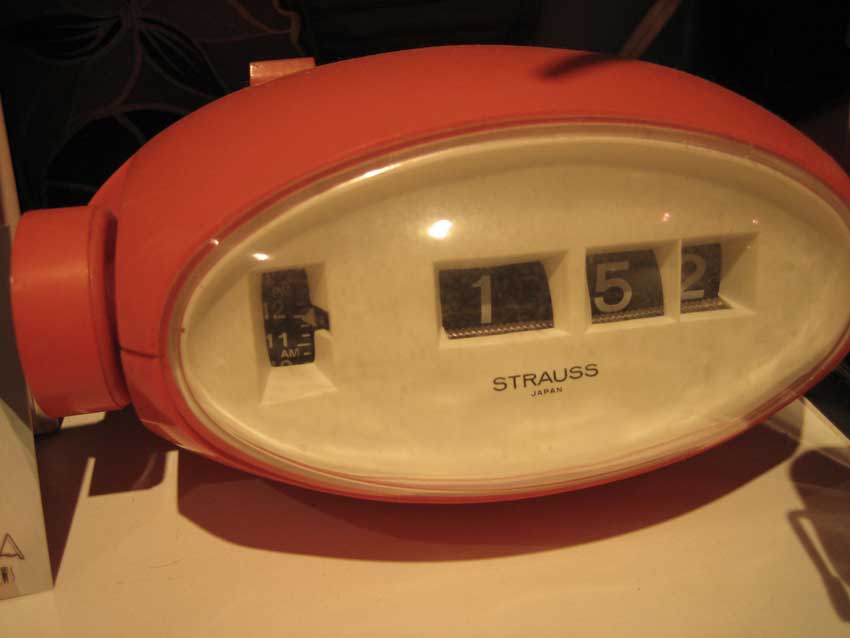This color photograph, taken inside a room with light casting shadows below, features a futuristic-looking Strauss clock made in Japan. The main object is an orange clock sitting on a smooth, white table, although the picture has a light brownish tint that slightly obscures the true color. The clock's design is reminiscent of a rocket, with an oval-shaped dial in front that displays the time as 1:52 in a retro flipping-page format, alongside other numbers like 12, 11, and designations like AM. The front of the clock also prominently features the brand name "Strauss" with "Japan" written below it. To the left of the main dial, there is a section showing a measurement at the 12 o'clock position. The background of the image includes a blend of brown, black, and gray tones, with some wood elements visible.